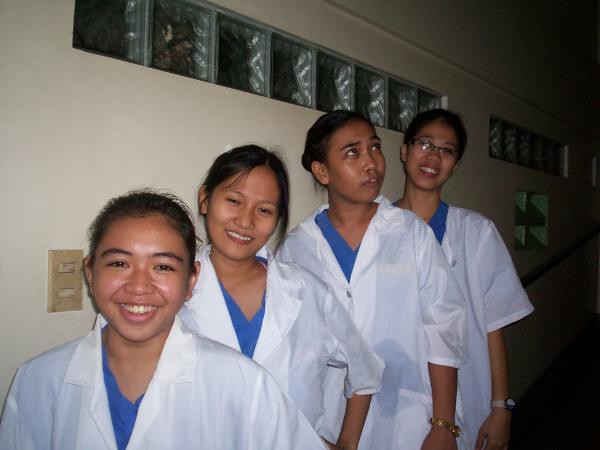This photograph captures four Asian women, likely medical professionals or students, standing against a white wall adorned with small square windows in a large rectangular frame. Arranged in ascending order of height, the shortest woman is at the front and the tallest at the back. Each one is donned in a white coat over dark blue scrubs, with the white fabric slightly see-through. 

The woman at the front, who is the shortest, is gazing directly at the camera with a smile. The second woman, a bit taller with longer black hair, shares a smile with the woman in front. The third woman, taller still, is making a goofy face as she looks up and to her left. The tallest woman in the back is wearing glasses and smiling directly at the camera. Notably, two of the women wear watches on their left wrists, though the details are unclear. One of the white coats appears to have a stain or wet spot.

The setting includes tan, dirty outlets on the wall and large windows segmented into smaller squares. Their collective demeanor is mostly cheerful, adding to the sense of camaraderie captured in this moment.